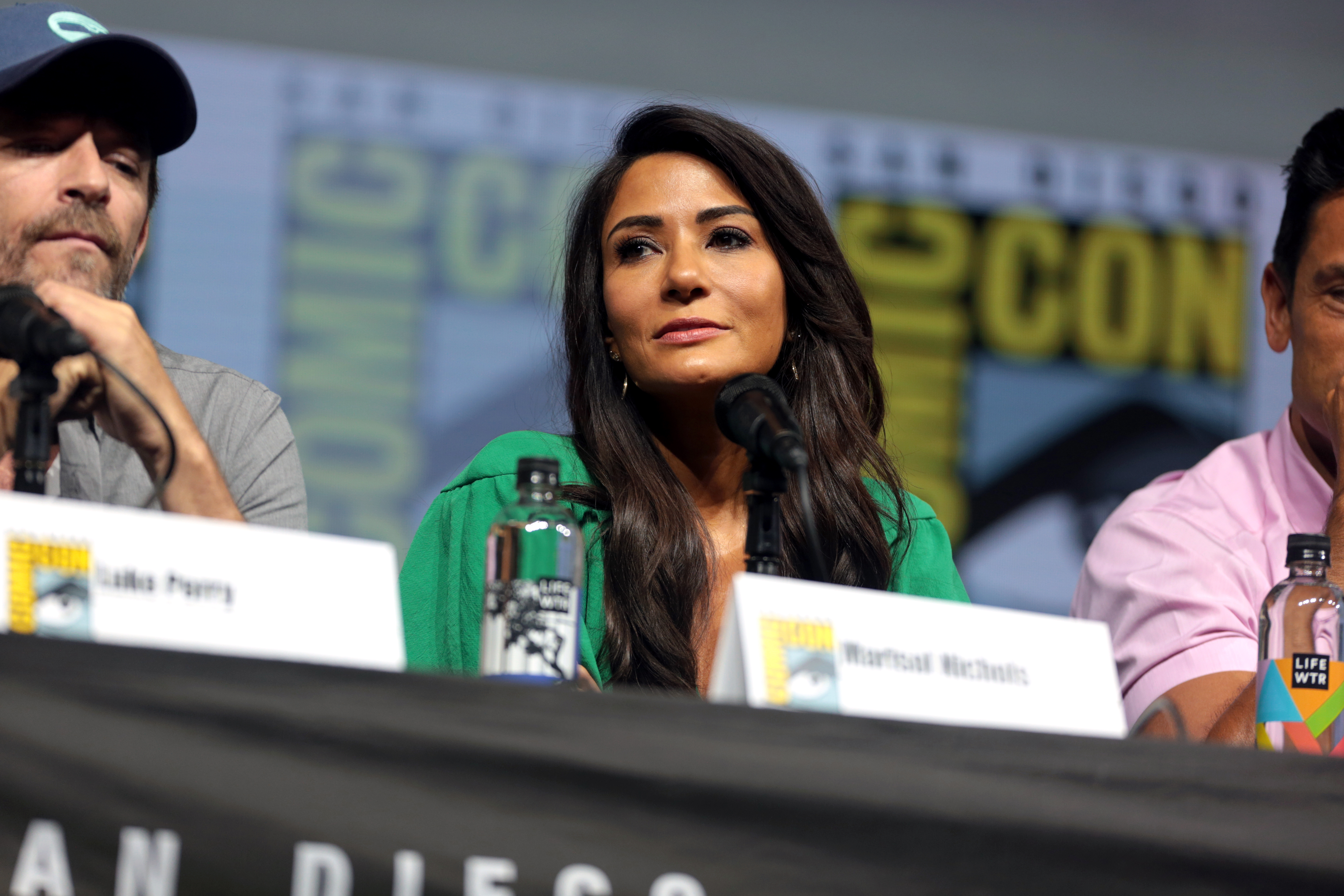This photograph, taken at a convention panel, features three people seated behind a table covered with a black tablecloth. In the center is a woman with long dark hair, dressed in a green shirt, with a black microphone positioned in front of her. To her left sits a man in a blue cap and gray t-shirt, who appears to be silent. On her right is another man, partially cropped out of the frame, wearing a pink shirt. The table is adorned with water bottles and name placards, although the names are blurred and illegible. The backdrop behind them is adorned with posters featuring the San Diego Comic-Con logo, with "San Diego" in black font and "Comic-Con" in bold yellow, set at an angle.